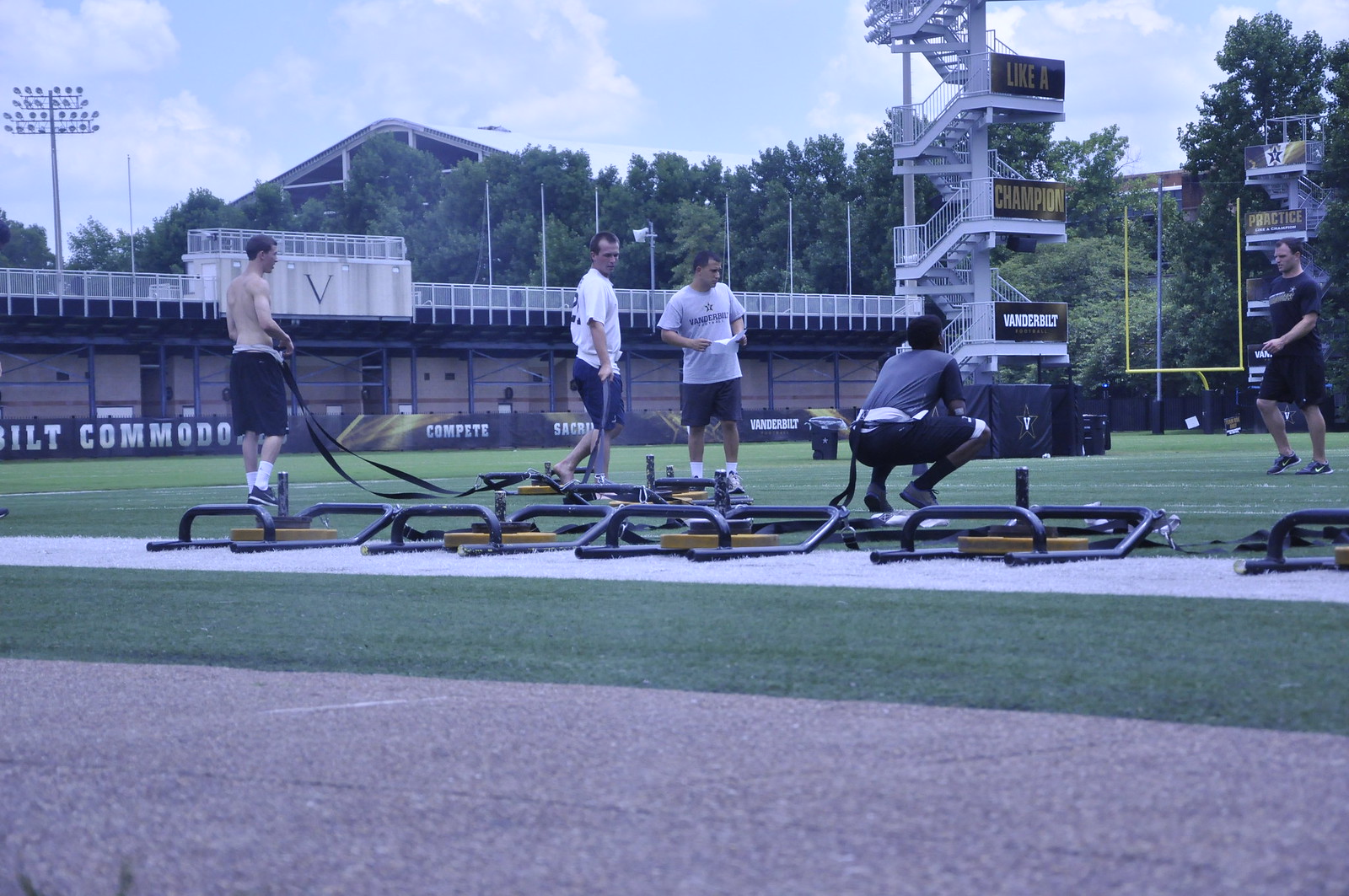The image showcases an outdoor football practice session at Vanderbilt University. The setting is a football stadium, characterized by a vibrant green artificial turf field with a distinct white line running across it. In the foreground, a paved track encircles the field. The background features a picturesque sky, blue with scattered white clouds, framed by a dense tree line comprising various trees including pines, oaks, and evergreens, which help obscure larger buildings and provide privacy.

On the field, five football players are engaged in a rigorous workout. One player is shirtless while the others are dressed in t-shirts, shorts, and Nike shoes. Each player wears a belt around their waist, attached to weights or sleds via visible straps. These sleds are likely loaded with weight plates to add resistance for their training exercises, aiming to enhance running speed and leg strength. One player is seen squatting, possibly between exercises, while the others stand around, suggesting a pause in their routine.

In the backdrop, a prominent steel staircase and a large banner with the words "like a champion Vanderbilt" are visible, alongside other banners and flags, adding to the collegiate atmosphere of the scene.